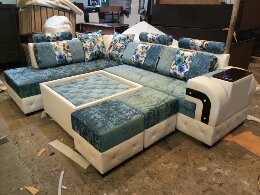This is an indoor color photograph featuring a sectional sofa with all pieces assembled to form a U-shape. The sofa, which looks dated and possibly from the late '80s or early '90s, showcases a color palette of light and dark blue with white accents. The patterns on the upholstery include denim and floral designs, while the bottom of the sofa and a matching brocaded poof in the center feature intricate brocade. The sofa has attached cushions along with round cylindrical pillows serving as headrests. Notably, the armrest on the left side features a small table on top of it. The sectional is situated on a concrete floor inside what appears to be a warehouse or storage facility, with other indistinct furniture visible in the background. Overall, the image captures a vintage, well-worn couch set that is likely on display.